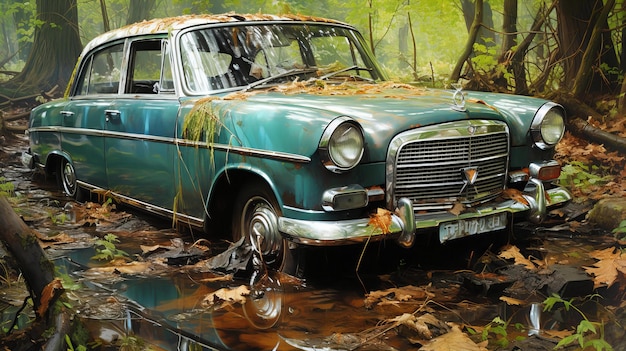In this up-close, highly detailed image of a classic teal and white antique car, the vehicle lies abandoned and half-sunk in a forest clearing, surrounded by water and decaying vegetation. The paint is a striking aqua blue with silver lines tracing the bumper, grille, and headlights. Despite its vivid colors, signs of age are evident; the white license plate is rusted and illegible, and the front right tire is buried halfway in the murky water. The car’s windshield reflects a stark white light, while its hood and roof are layered with brown dead leaves and some sprigs of green grass. The right window is notably rolled down, exposing the weathered interior. Around the vehicle, puddles of brown and blue water host floating leaves, indicative of the car's prolonged abandonment. Behind this scene, tree trunks pierce a misty backdrop, adding to the sense of desolation and timelessness.